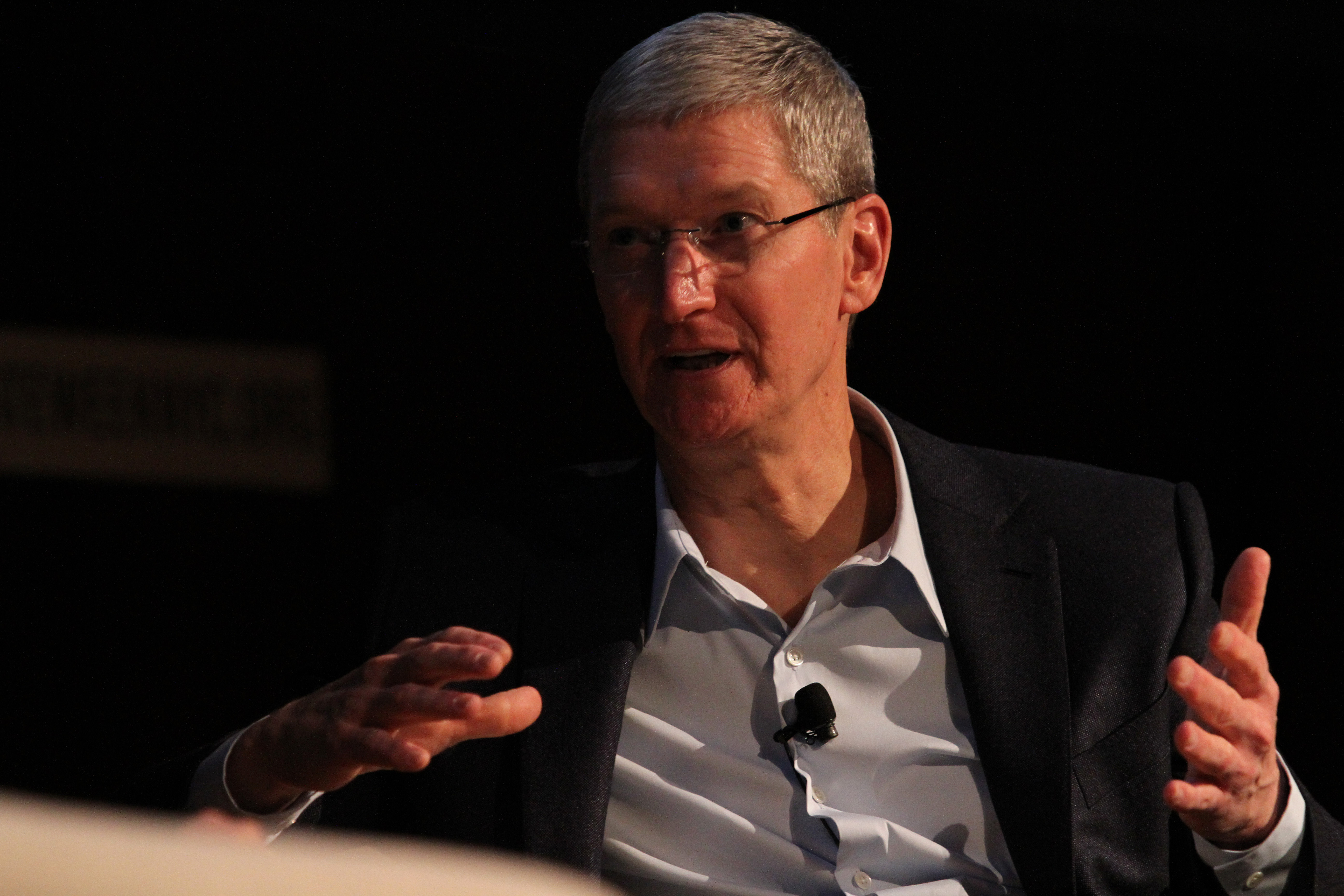The photograph features Tim Cook, the CEO of Apple, centered and seated at a table. He is a white male with short, silver-gray hair, and is wearing glasses with black frames. Cook is captured mid-conversation, his mouth open, and his gaze directed to the left. He's dressed in a black blazer over a light blue button-down collared shirt. A small black microphone is clipped to the center of his shirt. Both his arms are outstretched, gesturing as he speaks—one hand positioned to the bottom right and the other towards the bottom center. The background is predominantly black, with the right side of the photo illuminated, creating a stark contrast against the darker left side. There are some indistinct features in the background, including what appears to be a rectangular area with black letters on a white background to the middle left, and a slightly visible, out-of-focus, off-white or beige-colored object at the bottom left.